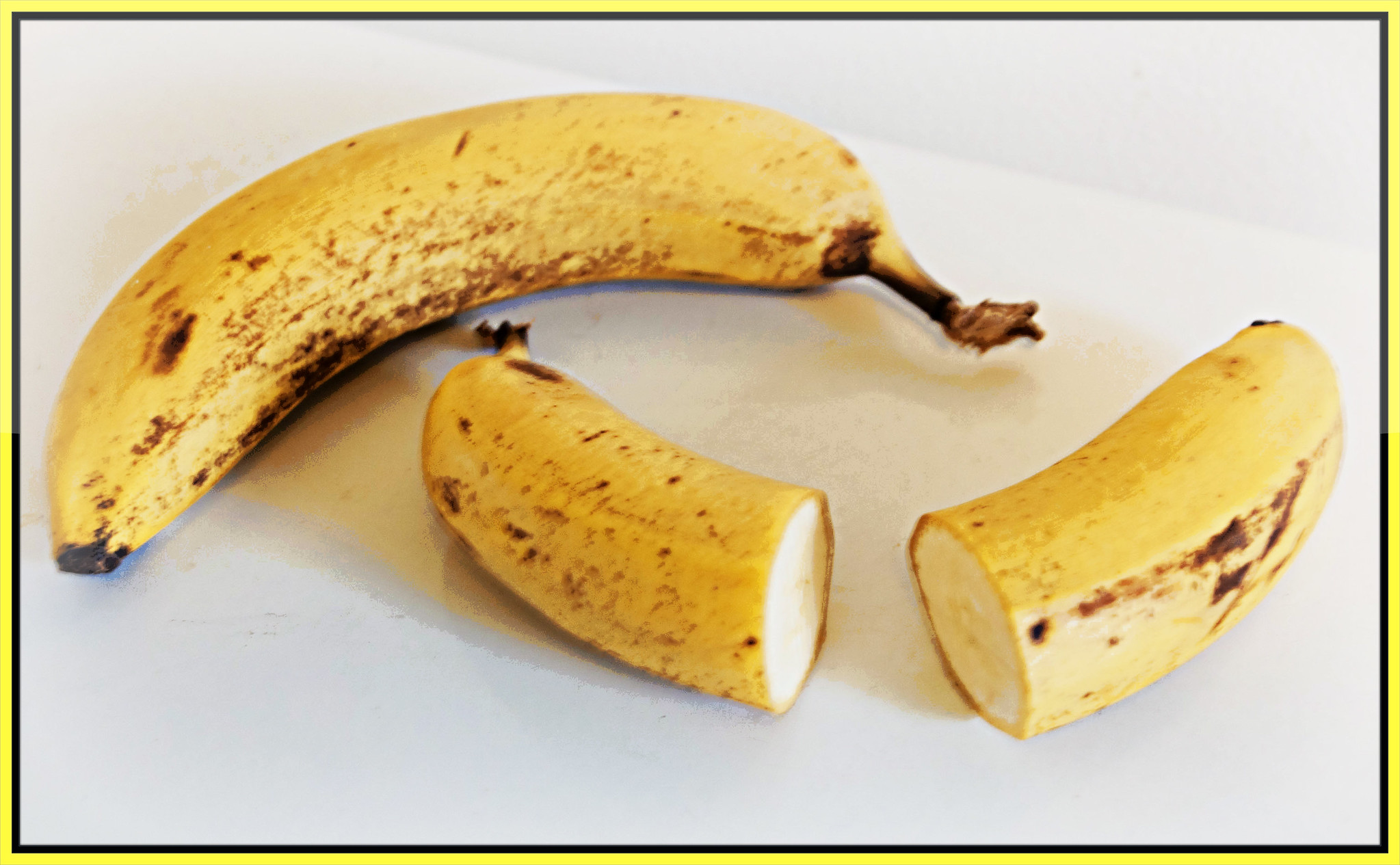This photograph features two bananas positioned on a plain, white table. The first banana, slightly browning, lies entirely curved away from the viewer. In juxtaposition, the second banana, similarly browned, mirrors the curvature of the first but is sliced in half, revealing its inner flesh from both halves. The composition is framed by a delicate black border, which is further accentuated by a thin yellow outer border, adding a touch of color contrast. The table is smooth and textureless, providing a stark, minimalist background that highlights the details of the bananas.